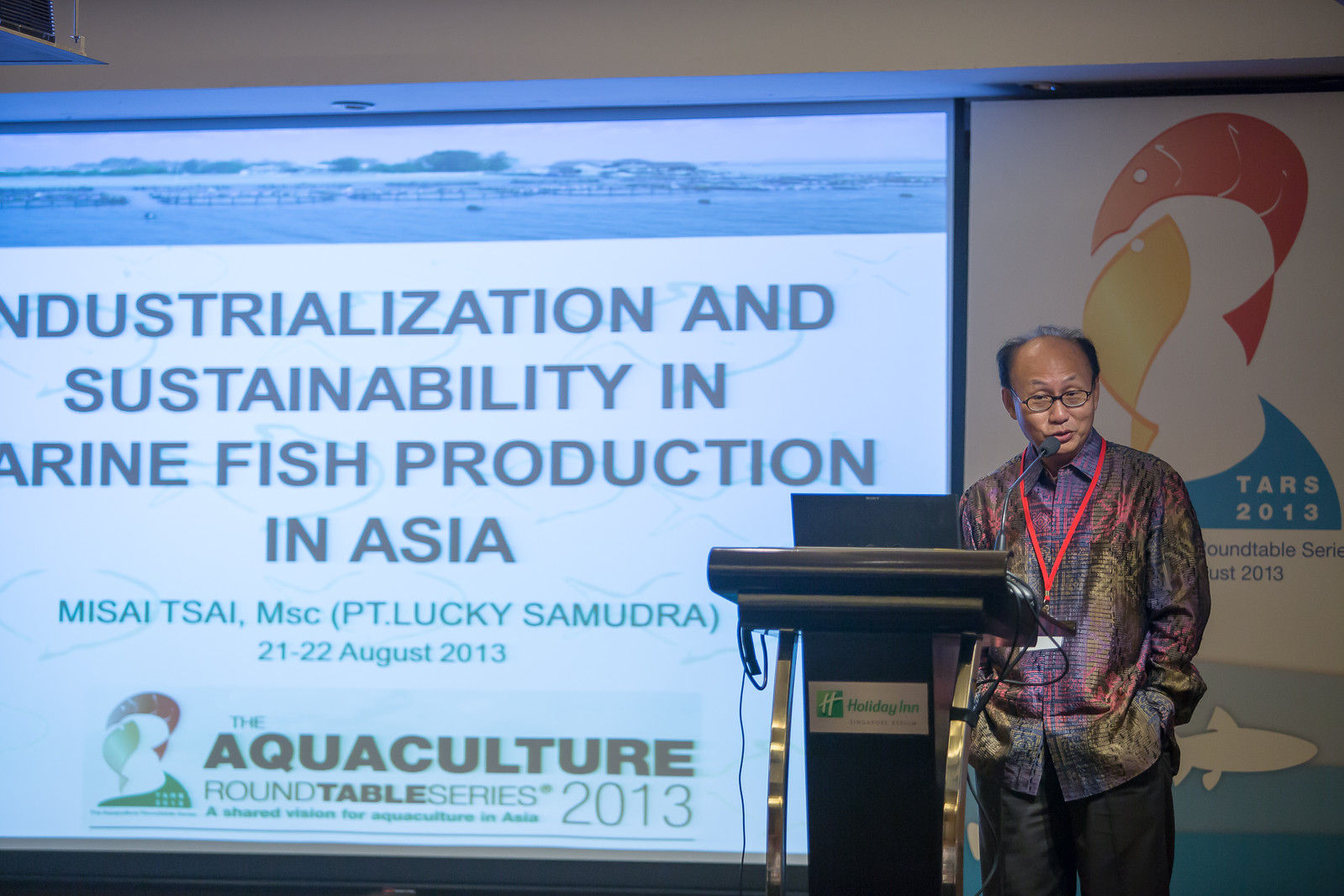The image depicts an older Asian man, likely in his 50s or 60s, delivering a presentation at a podium. He is wearing glasses, a multicolored dress shirt that gives off a vibrant and iridescent appearance, and plain pants. He has a receding hairline with short black hair on the sides and is speaking into a microphone. The podium features a sign reading "Holiday Inn Singapore," indicating the venue of the presentation. In the background, a large sign reads "TARS 2013," accompanied by a logo of two fish jumping out of water. To the left of the podium, a screen displays a slide titled "Industrialization and Sustainability in Marine Fish Production in Asia," with mentions of the Aquaculture Roundtable Series taking place from August 21st to 22nd, 2013. The slide also includes the text "P.T. Lucky Samudra" and a depiction of a marina.